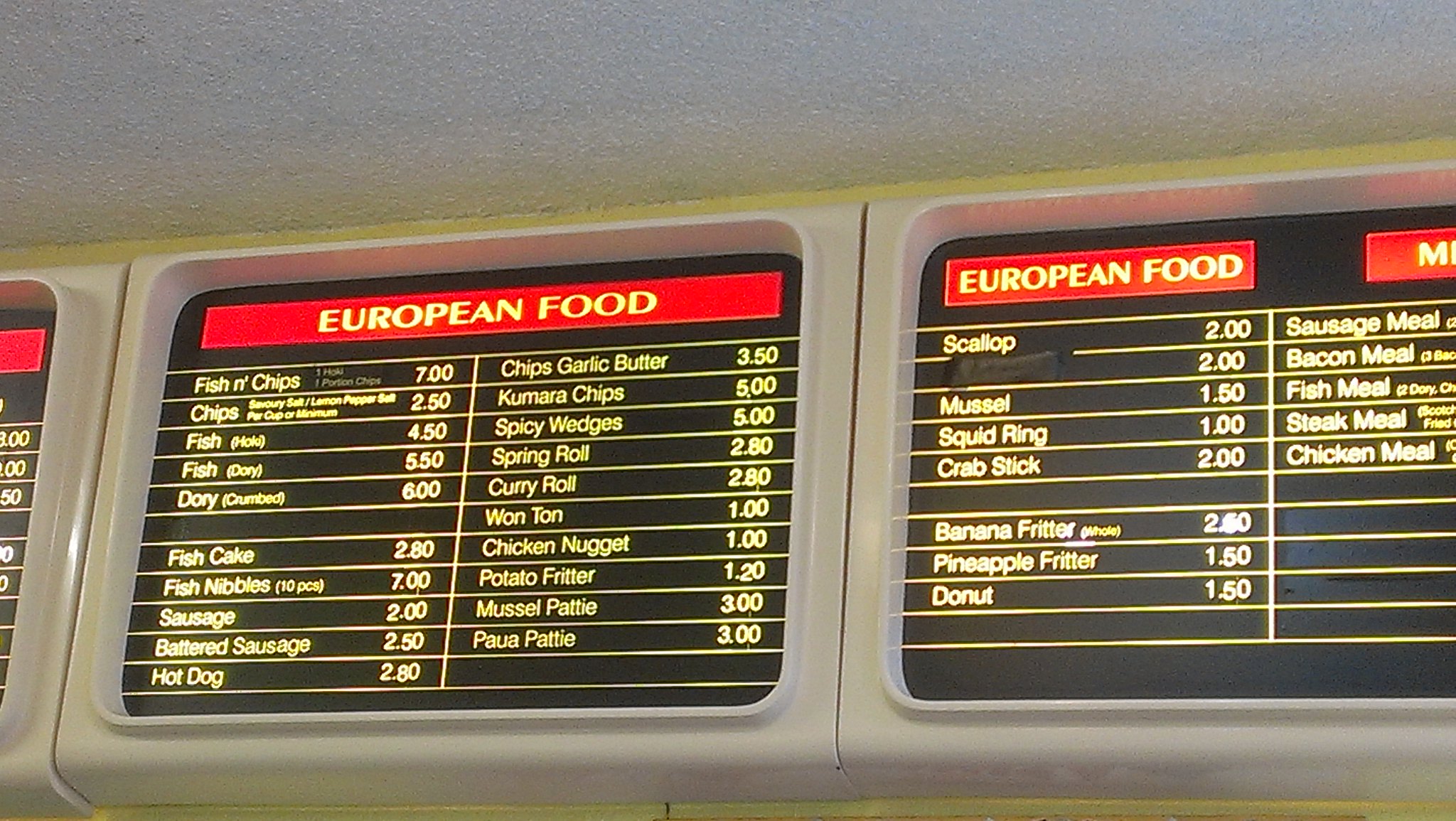A detailed description of a takeout menu at a restaurant is prominently displayed above the ordering desk, adjacent to the cash register. The menu features an eclectic assortment of items categorized under "European food," though the selection might seem somewhat random. 

Written in a striking yellow-gold font against a red background, the left side of the menu includes:

- Fish and chips priced at 7 units (the exact currency is unclear)
- A variety of chips
- Fish cakes and fish nibbles
- Sausages, including both traditional and battered versions
- Hot dogs

On the right-hand side, additional European food items are listed, equally affordable regardless of the unspecified currency. This section includes:

- Scallops
- Mussels
- Some items which are unreadable due to being whited out or blacked out
- Banana fritters

The display is mounted on a plastic gray base and is set against a yellowish wall. The ceiling above features a textured white surface, adding to the visual complexity of the setting.